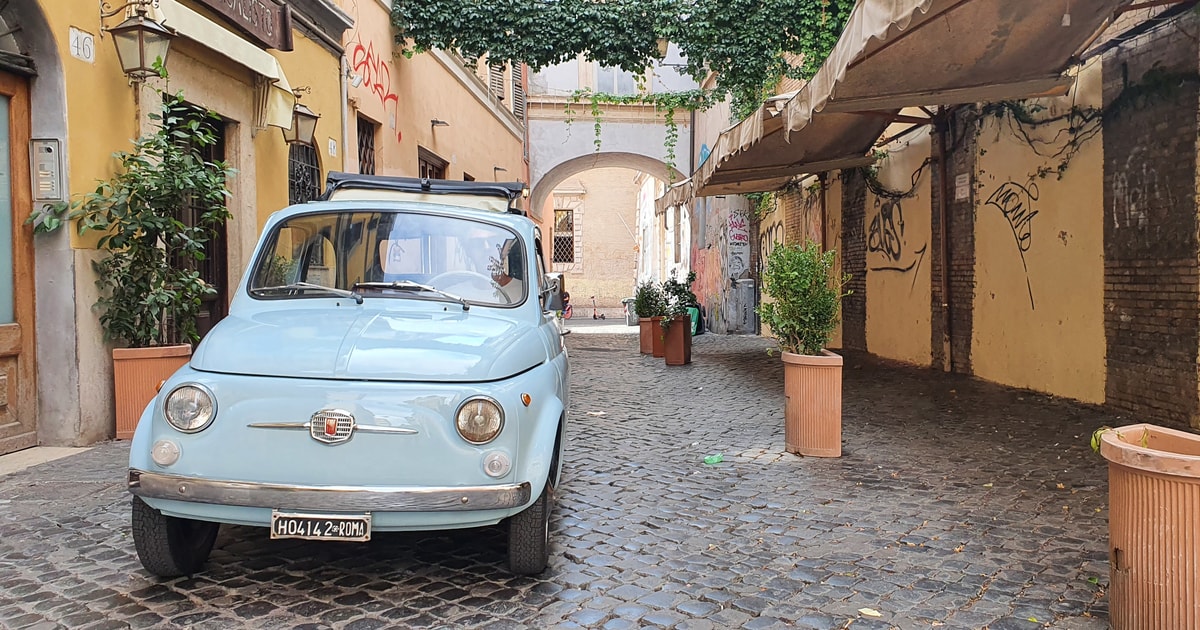The image is a vertically rectangular, full-color photograph taken outdoors during the daytime using natural light. It captures a charming, narrow cobblestone street. Dominating the scene is a light blue, classic-style car parked on the cobblestone road. The car has a European license plate reading "H04142 Roma" and features circular headlights and a red rectangular logo. 

To the left side of the car is a yellow stucco building marked with the number 46, featuring an arched doorway adorned with a light fixture and a potted tree positioned near the entrance. The building facade reveals another light and some red graffiti. Above the scene, at the center top of the photograph, you can see vines hanging down, adding to the quaint atmosphere. There's also an awninged area and another brown stucco building covered in black graffiti.

The image beautifully captures the interplay of light, casting reflections on the car and illuminating the picturesque alley flanked by buildings on either side. The overall ambiance is bright and serene, typical of a sunlit European street.